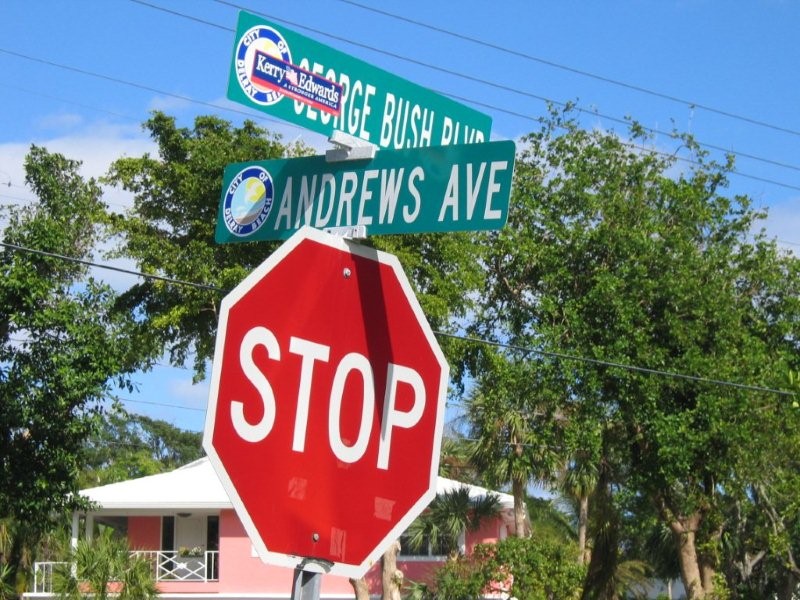On a sunny day with clear skies, the image captures a picturesque neighborhood scene with distant mountains and lush green trees. A striking pink house with a white roof and a white porch gate is visible, alongside several tropical palm trees, suggesting the location might be in California or Florida. Central to the image is a bright red stop sign with distinct white letters spelling S-T-O-P, outlined by a white border around its octagonal shape. Atop the stop sign, two green street signs point in opposite directions: the left sign reads “Andrew Zabin” in white text, and the right sign, partially obscured by a Carrie Edwards campaign sticker, reads “George Bush Drive” in white text.